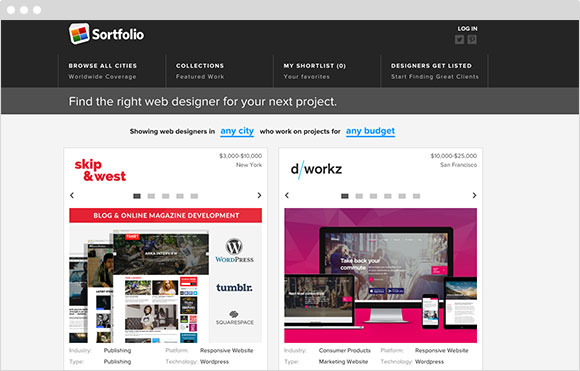In this image, we see a detailed view of the Sortfolio website's homepage. At the top left, the Sortfolio name is displayed alongside their logo, which resembles a piece of paper divided into four colored squares: orange, red, green, and blue. Moving to the top right corner, three small white circles are aligned horizontally. Just below these circles, in the top right section, the word "Login" appears in white text. Beneath this, there are two gray boxes containing social media icons for Twitter and Pinterest.

In the top-middle section of the page, four main navigation categories are listed from left to right: "Browse All Cities," "Collections," "My Short List," and "Designers Get Listed." Below these categories is a boxed area featuring a call-to-action text that reads, "Find the right designer for your next project."

Further down, in the center of the image, there are two boxed areas placed side by side. The box on the left contains the text "Skip and Wes" written in a red font, with five small squares below it. The first square is dark gray, and the remaining four are light gray. The box on the right is labeled "D Works" and also features five small squares below it in the same color scheme. This detailed layout provides an organized and visually clear representation of the Sortfolio website's homepage.